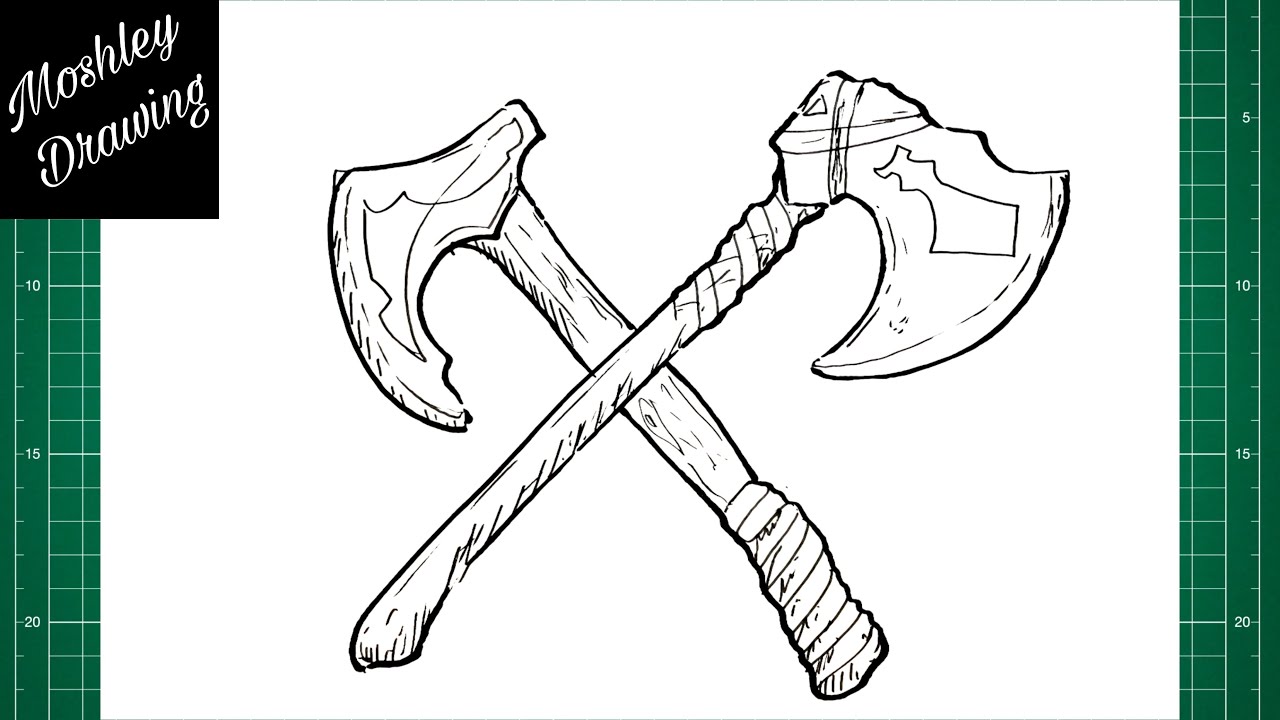The image is a horizontal graphic design in black and white, prominently featuring a central drawing of two vintage-style axes crossed in an 'X' formation. These axes, situated against a stark white background, are rendered in detailed black ink. The axe that extends from the lower right to the upper left has a wooden handle wrapped in fabric for added grip, while the other, crossing from the bottom left to the top right, features its handle wrapping closer to the blade. Both axes have long, curved blades, slightly widening at the tips.

In the top left corner of the design is a black square with cursive text in white reading "Moshley Drawing." Behind the main image, to both the left and right sides, a cutting board or drafting grid can be seen. This background grid is green with white lines and labeled hash marks running along the edges, numbered at intervals—creating a measuring backdrop that highlights the axes' size and intricate details. The entire composition showcases a blend of traditional and digital art elements, emphasizing the meticulous craftsmanship involved.